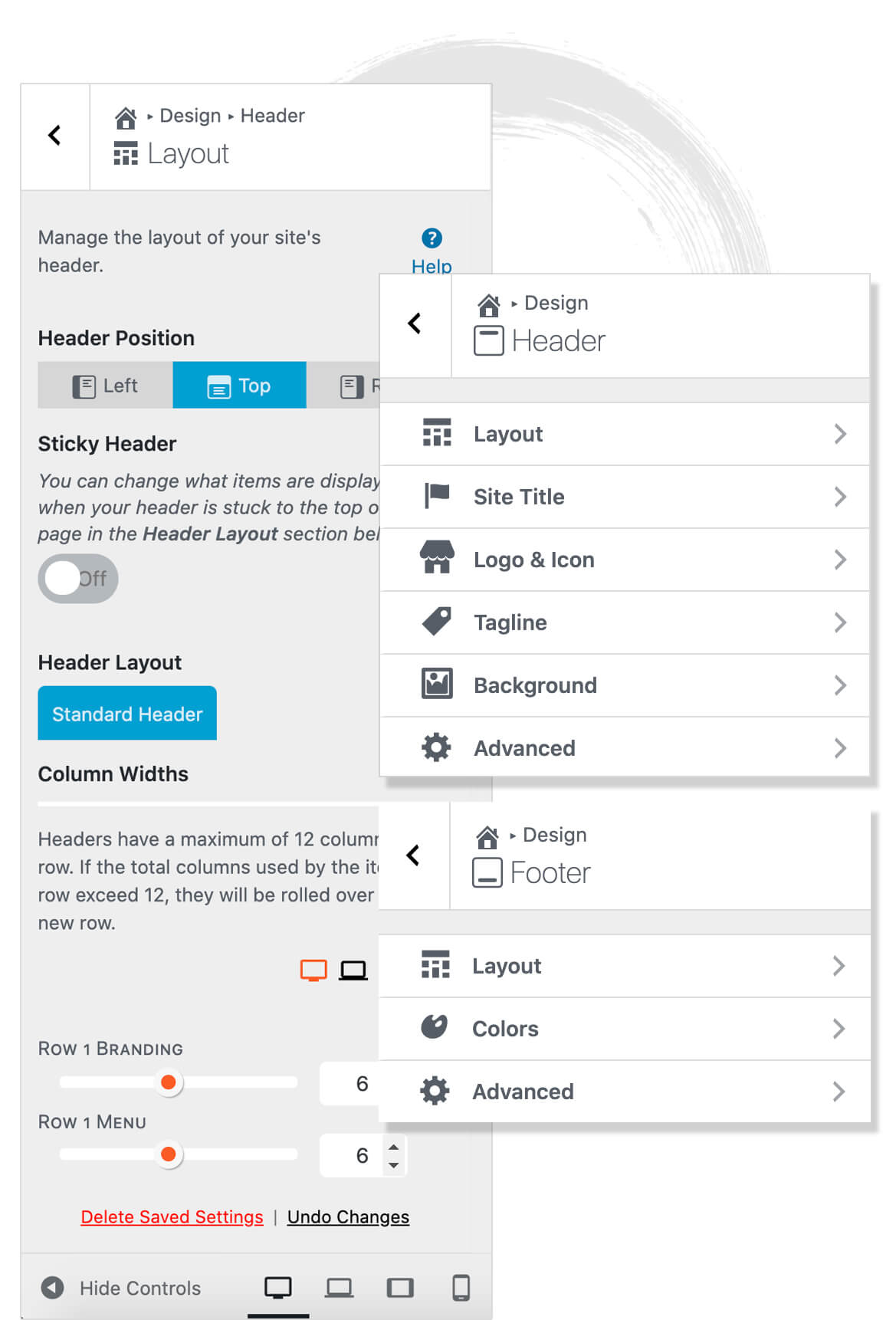**Detailed Description of Two Overlapping Dialog Boxes:**

In the image, there are two dialog boxes with the second one partially overlapping the first. 

The first dialog box, positioned on the left side of the image, measures approximately 12 inches in length and 3 inches in width. Its primary background is a gray shade, with black font and headers. At the very top, a white section contains the title "Design Header Layout". Underneath, a series of configurable options related to the site’s header layout is available. 

- **Header Position:** Users can select the header position (left, top, or right), with the "top" position currently highlighted in blue, indicating it's the active selection.
- **Sticky Header:** Only three-quarters of this section are visible, but it instructs that you can change the items displayed when the header is stuck to the top of the page. This option appears toggled off.
- **Header Layout Options:**
  - **Standard Header Column Widths:** Headers can use up to 12 columns per row. If the total exceeds 12, they will presumably roll over to a new row, although not all text is visible.
  - **Row 1 Branding Selection:** Includes a slider ranging from 1 to 10, currently set at 6.
  - **Row 1 Menu:** Similarly, features a slider from 1 to 10, also set at 6.
  - **Options for Deleting Sub-saved Settings or Undoing Changes.**

The second dialog box, which is in the foreground and slightly overlapping the first, is offset to the right and measures around 6-7 inches in length and 4 inches in width.

- **Design Header:** At the top, the title "Design Header" is displayed.
  - **Layout Options:** Including Site Title, Logo and Icon, Tagline, Background, and Advanced Settings. An arrow next to each option indicates that clicking will reveal further configurable settings.
  - **Design Footer:** Below the header section, there are options to design the footer, with settings for Layout, Colors, and Advanced Options.

This detailed description provides a comprehensive overview of the dialog boxes, their measurements, and the various configurable options they offer.